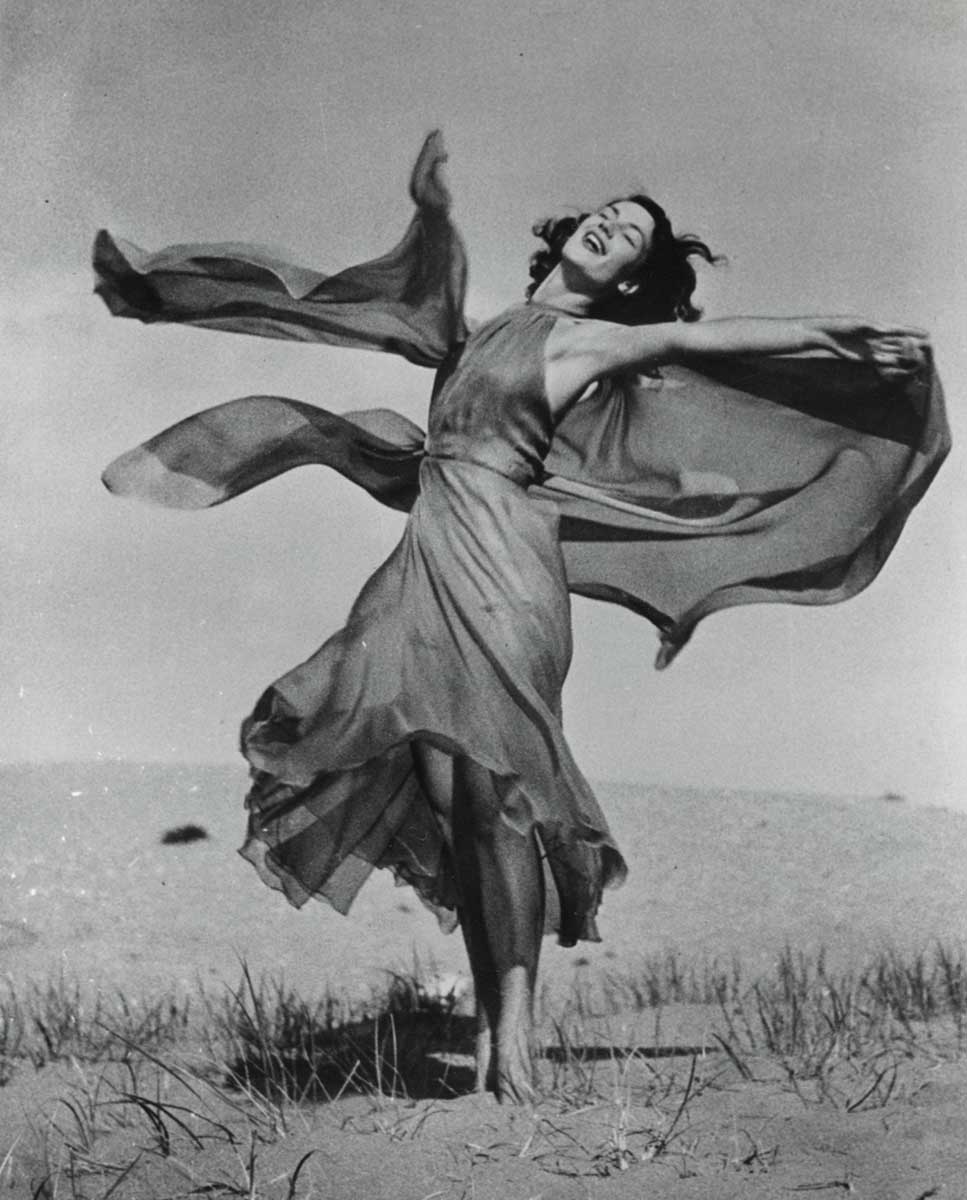This black and white photograph captures a moment of pure joy and freedom featuring a woman in a large, flowy dress. The dress, possibly made of a satiny fabric, extends from just below her knees up to her chest and billows dramatically around her as she twirls, her movements suggesting the grace of a ballerina. She stands barefoot in a grassy field, with the sky taking up about three-quarters of the background, giving an impression of open space and a touch of wilderness. Her left arm is extended, grasping the fabric of her dress, while her right arm seems to be hidden behind the flowing material, adding to the dynamic energy of the scene. Her dark hair, caught in motion, falls back as her head tilts backward in what can only be described as a moment of bliss, her eyes closed and a carefree smile gracing her face. While the photograph is devoid of color, the setting could be mistaken for a beach near water, adding a layer of ambiguity and intrigue to the picture. The slight undulation in the terrain and springs of grass allude to the natural beauty of the location, making the image a harmonious blend of elegance and spontaneous joy.